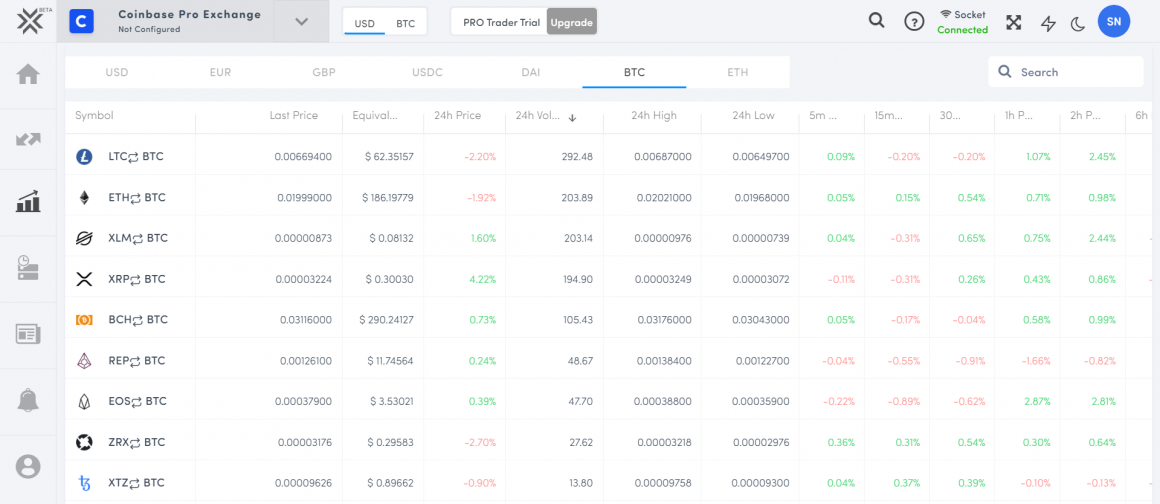The screenshot displays the Coinbase Pro Exchange interface, which is currently not configured. At the top left corner, there's a "Beta" label with two "V" shapes forming a cross-like symbol. 

Below the "Beta" label, there are several icons: 
1. A house representing "Home."
2. Two arrows pointing in opposite directions, potentially indicating "Transfer."
3. Bars with an accompanying arrow, suggesting a market or trading view.
4. A list with bullet points.
5. A clock icon.
6. A piece of paper icon.
7. A bell icon.
8. A user icon.

Underneath these icons, the trading pairs section highlights USD trading pairs, with BTC underscored in blue, indicating Bitcoin is selected. The phrase "Pro Trader Trial Upgrade" appears nearby.

Further down, the exchange lists different currencies: USD, EUR, GBP, USDC, DAI, with BTC underlined in blue again.

The trading data header includes columns for:
- Symbol
- Last Price
- Equivalent (likely abbreviated)
- 24-hour Price
- 24-hour Volume
- 24-hour High
- 24-hour Low

Time intervals for price data are also displayed: 5-minute, 15-minute, 30-minute, 1-hour, 2-hour, and 6-hour charts. The main part of the screen appears to be a chart displaying the selected market data.

The entire layout showcases a comprehensive trading dashboard, detailing multiple aspects of cryptocurrency trading on Coinbase Pro.